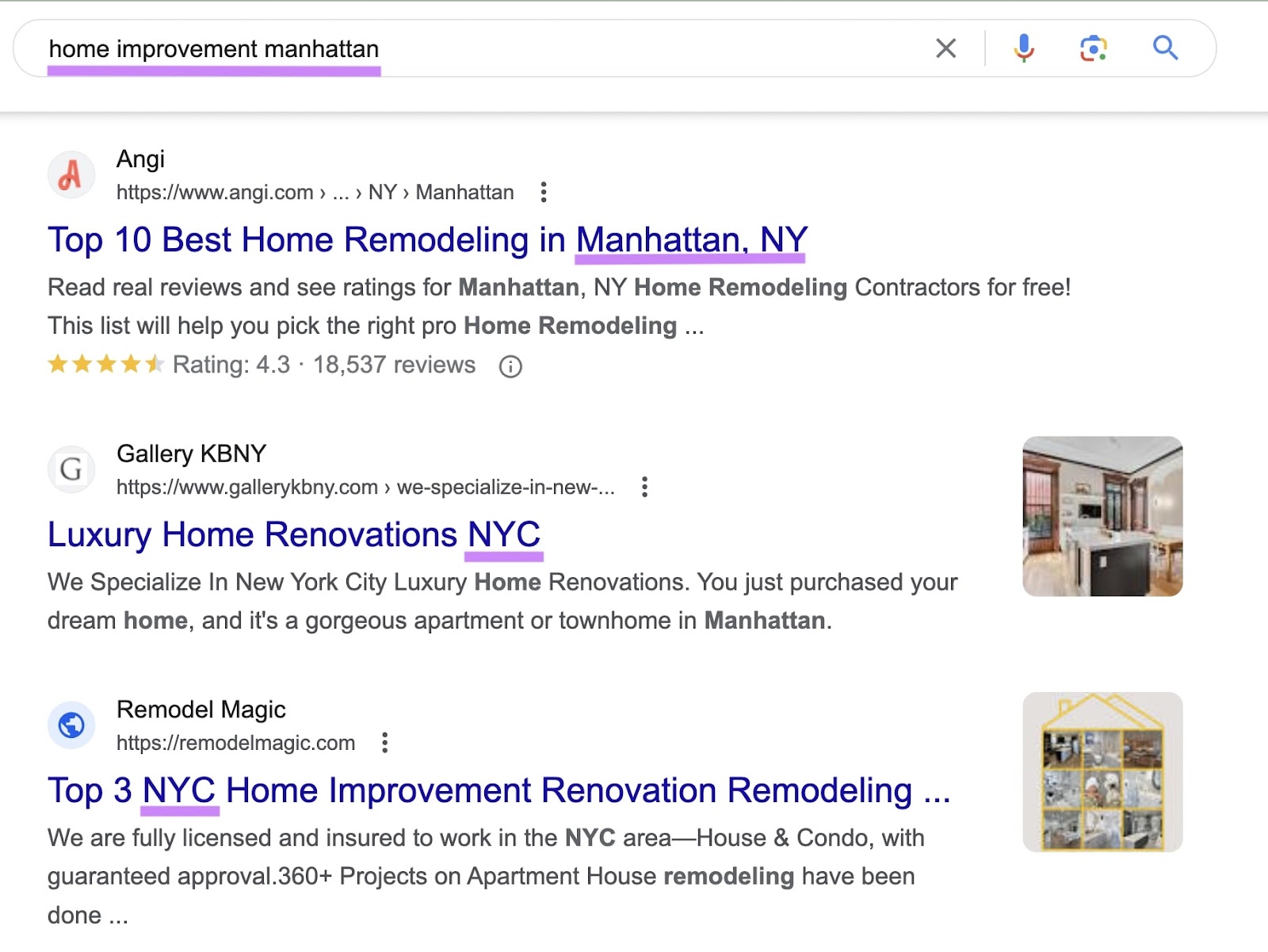The image depicts a search results page for home improvement services in Manhattan. At the very top, a bar in purple reads "Home Improvement Manhattan," which is followed by navigational icons including an 'x' to exit, a microphone, and a photo icon, suggesting it might be a voice or photo-based search tool.

The first result is for a service named "Adjie," identified by a red 'A' icon. It highlights "Top 10 Best Home Remodeling in Manhattan, New York," and encourages potential clients to read real reviews to see ratings for home remodeling contractors. The service boasts an average rating of 4.3 based on 18,537 reviews.

Below that, "Gallery KBNC" offers luxury home renovations in New York City, specializing in high-end projects for apartments and townhouses in Manhattan. The description paints a picture of moving into a dream home that has been expertly remodeled.

The next result, "Remodeled Magic," claims to be one of the top three home improvement and renovation services in New York City. The company is described as fully licensed and insured, with a portfolio boasting over 360 completed projects on apartments and houses. They guarantee approval for their work, which encompasses a variety of renovation needs.

Notably, the last two entries in the search results include images to the left of their text descriptions, adding a visual element to their listings.